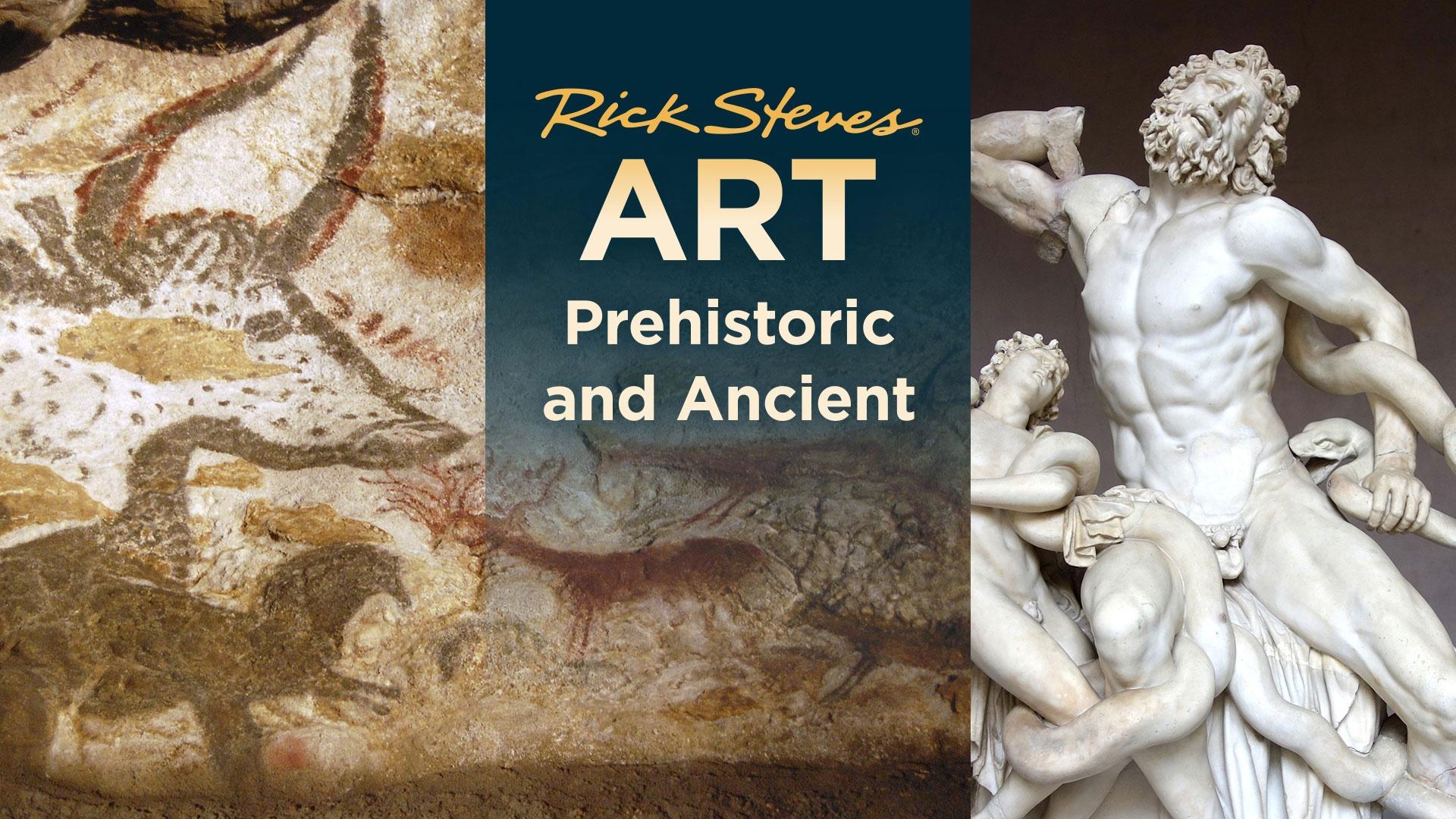The image showcases a promotional advertisement for an art museum event featuring "Rick Steves: Art Prehistoric and Ancient." Divided into two distinct sections, the left side displays a tan or light brown background resembling rock, adorned with various prehistoric engravings and cave paintings. These artworks include depictions of animals like horses, deer, and possibly dinosaurs, created with brownish paint on a white stone surface.

The center of the image contains a vertically oriented, transparent banner with a dark greenish-blue hue at the top that fades to clear at the bottom. The banner prominently features the event details: "Rick Steves" in elegant gold script, followed by "art prehistoric and ancient" in capitalized white font.

On the right side, a detailed marble or stone carving from ancient Greek or Roman times is depicted. The main figure is a contorted man seated on a chair, gripping a snake in his left hand while his right hand is curled toward his shoulder. Surrounding him is another smaller figure, possibly a woman, adding to the drama of the scene. The colors in the image span a palette of gray, black, light yellow, light orange, light brown, dark brown, off-white, and dark blue, enhancing its visual appeal. This digitally created composition blends real photos and striking artwork to effectively promote the museum event.